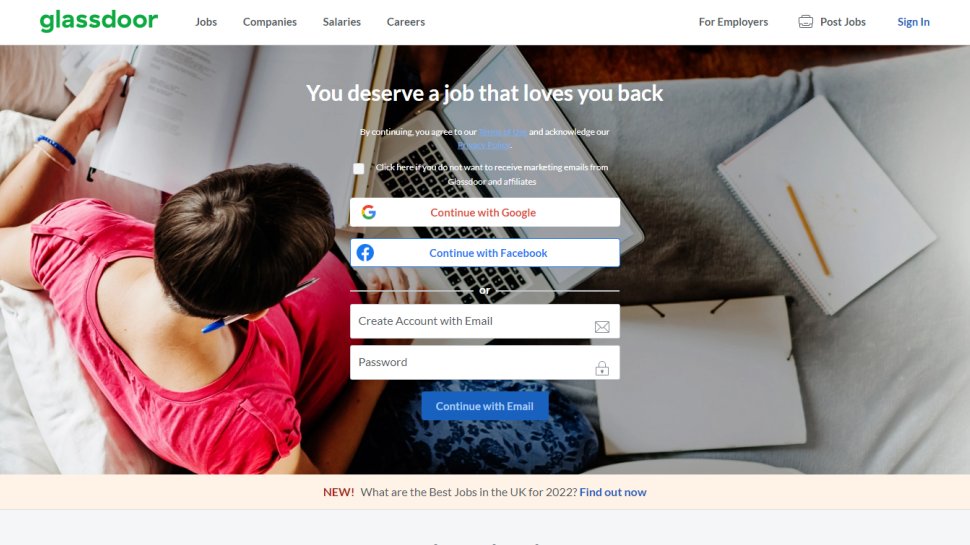This image features a digital interface overlaid on a rectangular area. At the very top, there is a green label reading "Glassdoor." Next to this, extending from left to right, is a string of black text ending with blue text, listing categories as follows: Jobs, Companies, Salaries, Careers, For Employers, Post Jobs, Sign In.

On the left side of the image is a woman with short black hair wearing a red shirt. She is seated either on a couch or a bed with several pillows behind her. The woman holds a book in one hand and rests a laptop on her lap, with her right hand on the keyboard. Additionally, she has a pen tucked behind her ear, capped in blue.

Centrally placed within the rectangle are large white letters proclaiming, "You deserve a job that loves you back." Under this text, there are smaller, less visible writings in white and blue. Below this, there are two white rectangles: the first has a Google logo with the text "Continue with Google" in blue, and the second contains a Facebook icon with the text "Continue with Facebook."

Further down, there is a dividing line followed by the word "OR," set between two more lines. Below this section, there are two additional rectangles labeled "Create account with email" and "Password." At the bottom, there is a blue rectangle with the text "Continue with email."

To the right side of the woman, a part of the couch or mattress is visible, with a paper spiral notebook lying alongside it, a pencil placed across the notebook. Next to the notebook lies another white piece of paper. The woman also wears navy blue pants speckled with black patches.